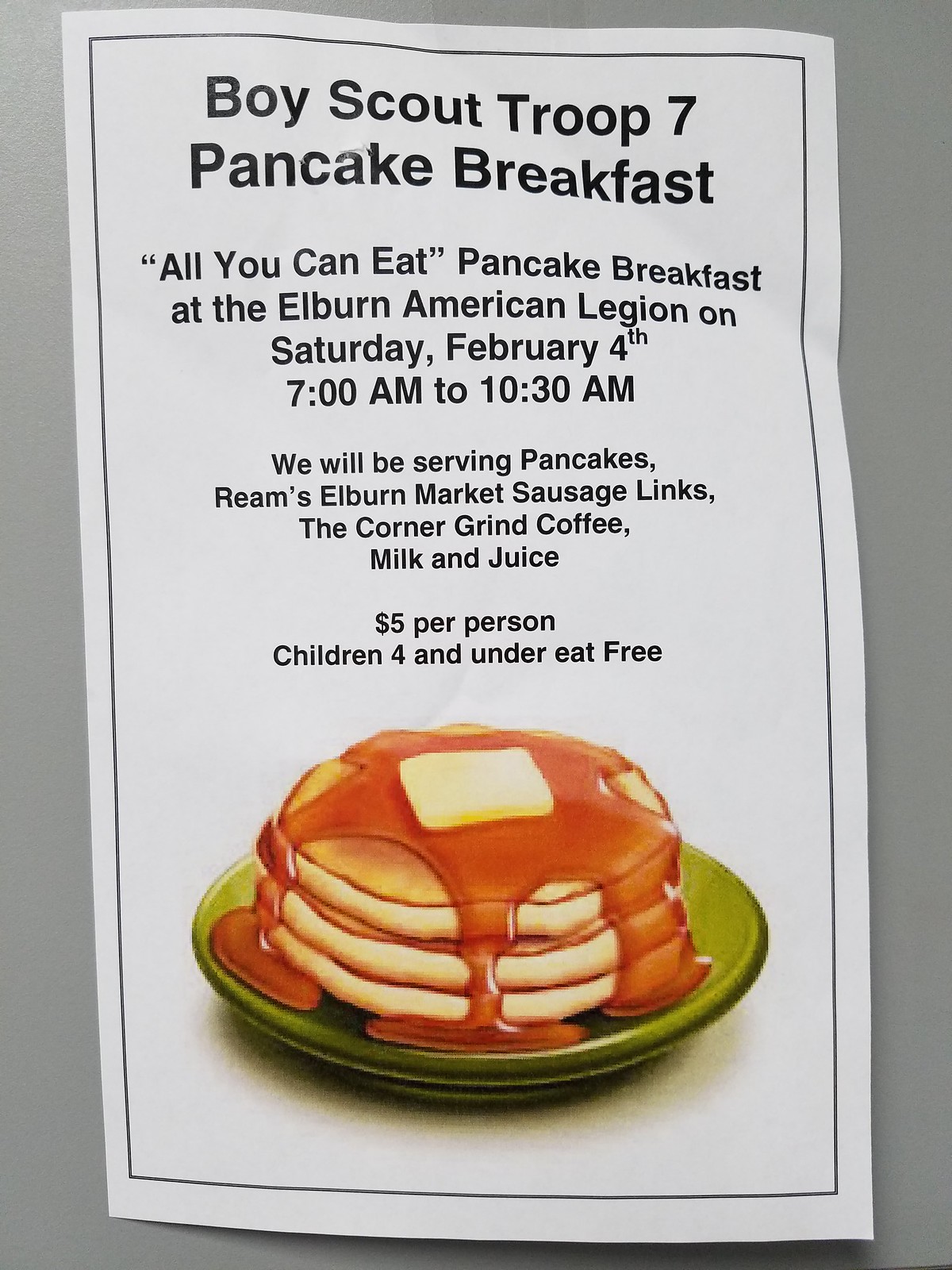This image features a flyer printed on white paper with a thin black border, posted against a gray surface. The flyer promotes the Boy Scout Troop 7 Pancake Breakfast, prominently displayed at the top in bold text. Below, it advertises an "all you can eat" pancake breakfast at the Elburn American Legion, scheduled for Saturday, February 4th, from 7 a.m. to 10:30 a.m. The flyer details the menu items, including pancakes, Reams Elburn Market sausage links, The Corner Grind Coffee, milk, and juice. It states the cost as $5 per person, with children aged 4 and under eating for free. At the bottom, there is an image of a green plate holding a stack of three pancakes, topped with a square pat of butter and generously drizzled with syrup that flows over the sides, pooling at the bottom.